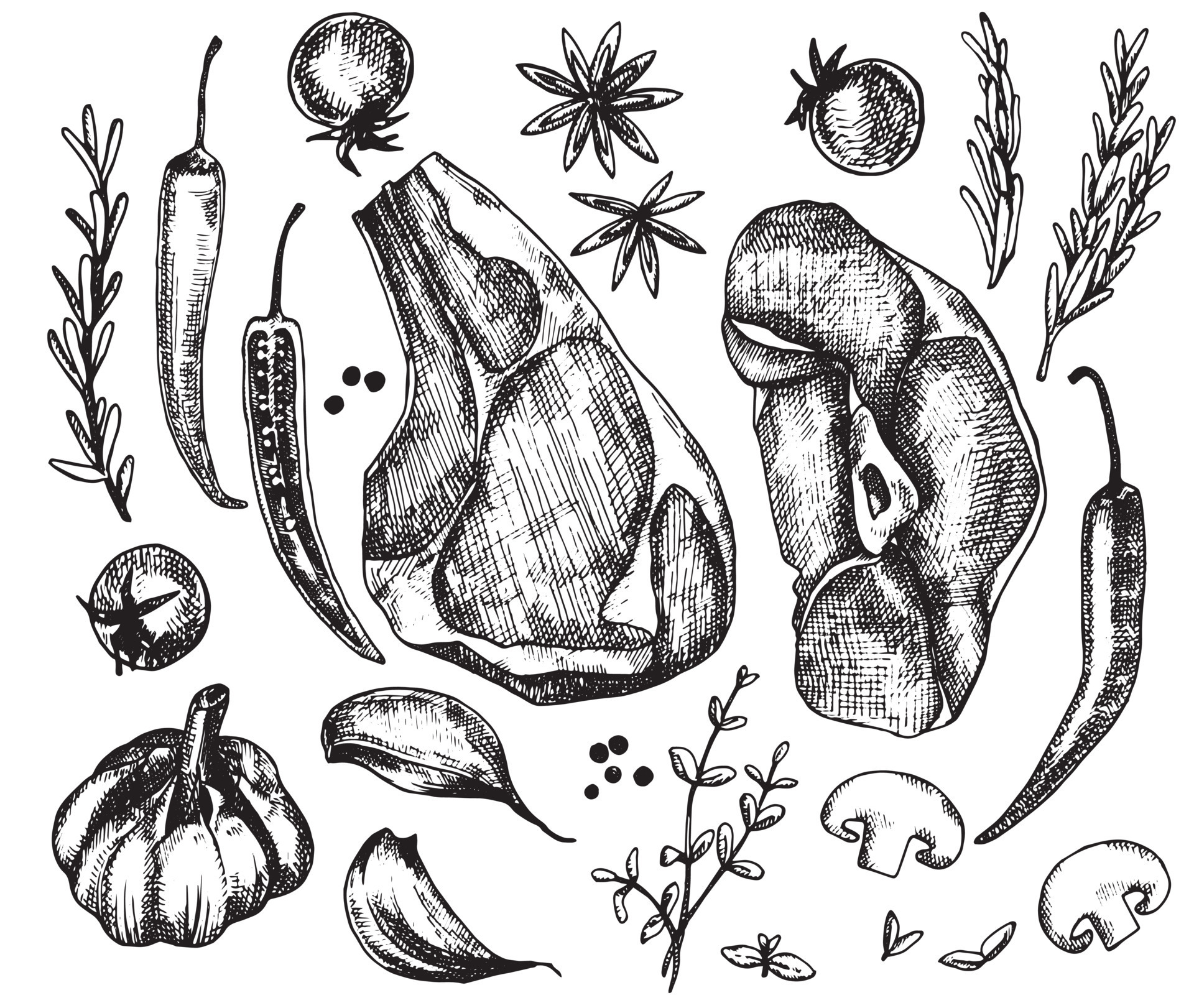The image is a detailed grayscale drawing, created in a style resembling hand-drawn art, which features an array of various food ingredients carefully laid out on a white background. Among the items identified are two pork chops prominently placed in the center. Surrounding the chops are several other ingredients: a split chili pepper and an unsplit chili pepper, star anise, a couple of cherry tomatoes scattered around, sprigs of rosemary and thyme, an entire head of garlic accompanied by two separate cloves, and sliced mushrooms. Also detailed are peppercorns, which are likely the "seeds" mentioned. Among the herbs included, there are also leaves, presumably from the thyme sprigs, sometimes mistaken for a bug from the distance. The overall composition is very orderly, depicting each ingredient with fine details and shadowing to enhance the monochromatic aesthetic.